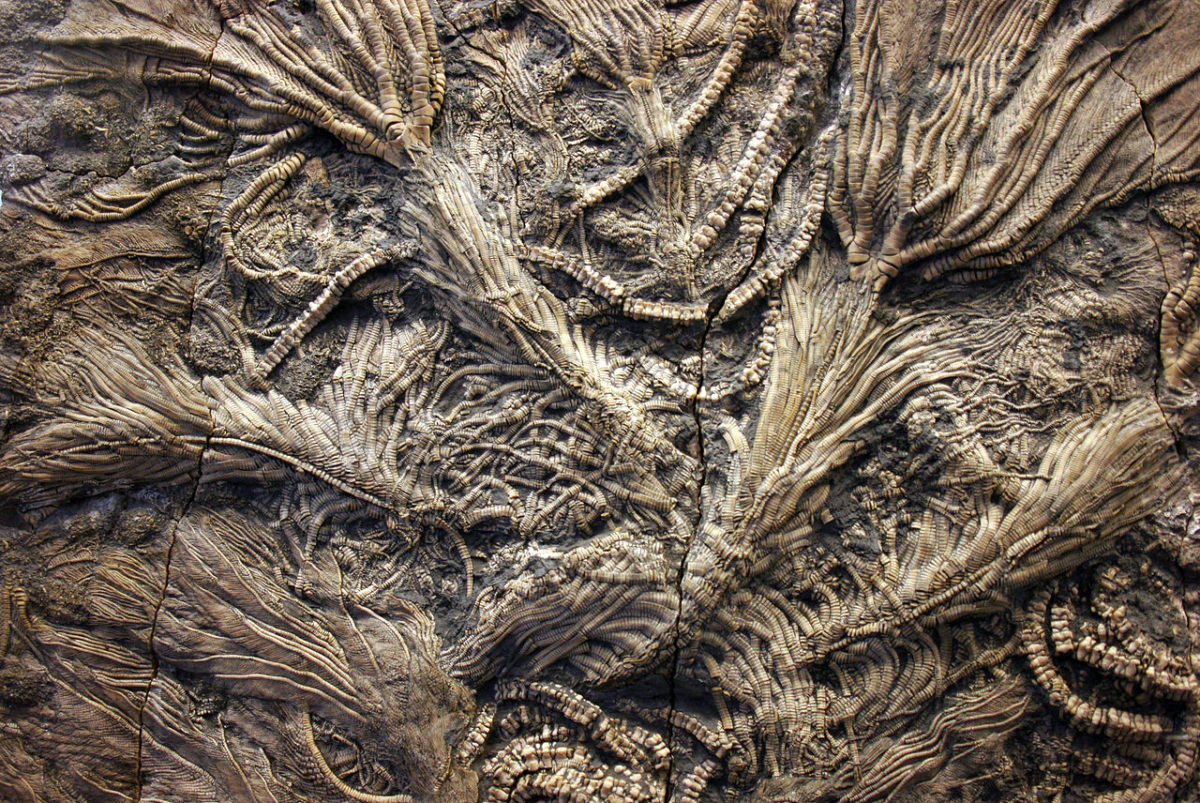This close-up photograph, likely taken outdoors in bright light, captures a dilapidated rectangle of textured material that appears old and weathered. The tactile surface features an intricate, jumbled arrangement of cloth remnants and perhaps even old feathers or stringy elements, all in a uniform gold, bronzy-beige color palette. Resembling beads, cobs, or roots, the interconnected pieces form rows and coils that enhance its complexity. Despite its natural appearance, this composition of random rags and decayed threads does not resemble living or plant forms, but instead evokes an image of decaying fabrics mingling together into a beautifully intricate tapestry.